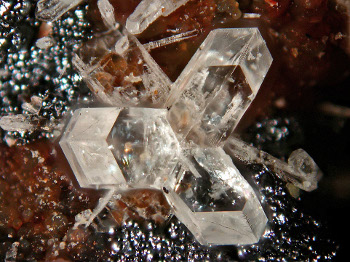The image depicts a small, super zoomed-in scene featuring several clear crystals that vary in shape and structure. Some of them resemble icicles or multifaceted diamonds, while one in particular has a distinct angel-like form with wing-like extensions that transition from cloudy at the base to clearer as they rise, revealing splashes of green, yellow, blue, gray, and pink within. Surrounding the crystals are numerous small, metallic silver and black beads or globes, scattered about in clusters. The background consists of an intriguing combination of brown, orange, tan, and black textures, which might resemble a rocky surface. Some areas also present a gummy brownish-orange texture. The composition is both intricate and mysterious, with varying textures and colors contributing to a captivating visual complexity.